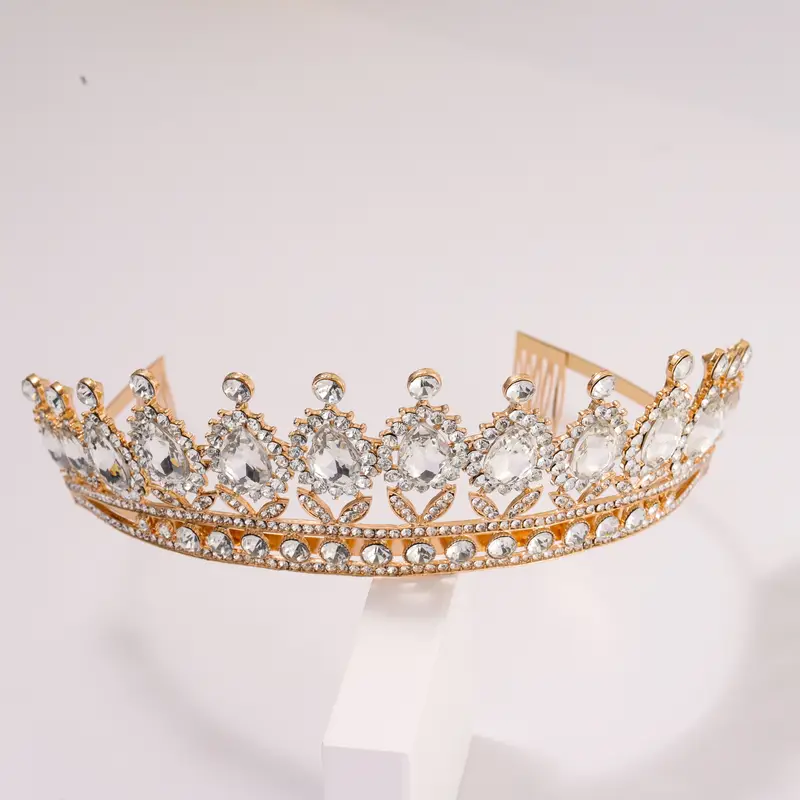This stunning rose gold tiara, displayed on a white brick stand against a solid white background, features an intricately detailed design adorned with clear, sparkling gemstones. The tiara nearly forms a complete circle, with small hair combs on each side at the back to secure it to the wearer’s head. Along the bottom of the tiara runs a continuous line of round, clear gemstones, flanked by smaller stones above and below. Rising from this base, the tiara showcases ornate leaf motifs filled with clear, shining stones. Crowning these motifs are very large, clear gemstones, each topped with a slightly smaller stone similar to those on the band. The gold elements of the tiara are predominantly hidden under the abundance of embedded gemstones, except on the backside where less decoration is present. This intricate piece evokes a sense of elegance and craftsmanship, making it appear almost regal, yet distinctly a tiara rather than a full crown.